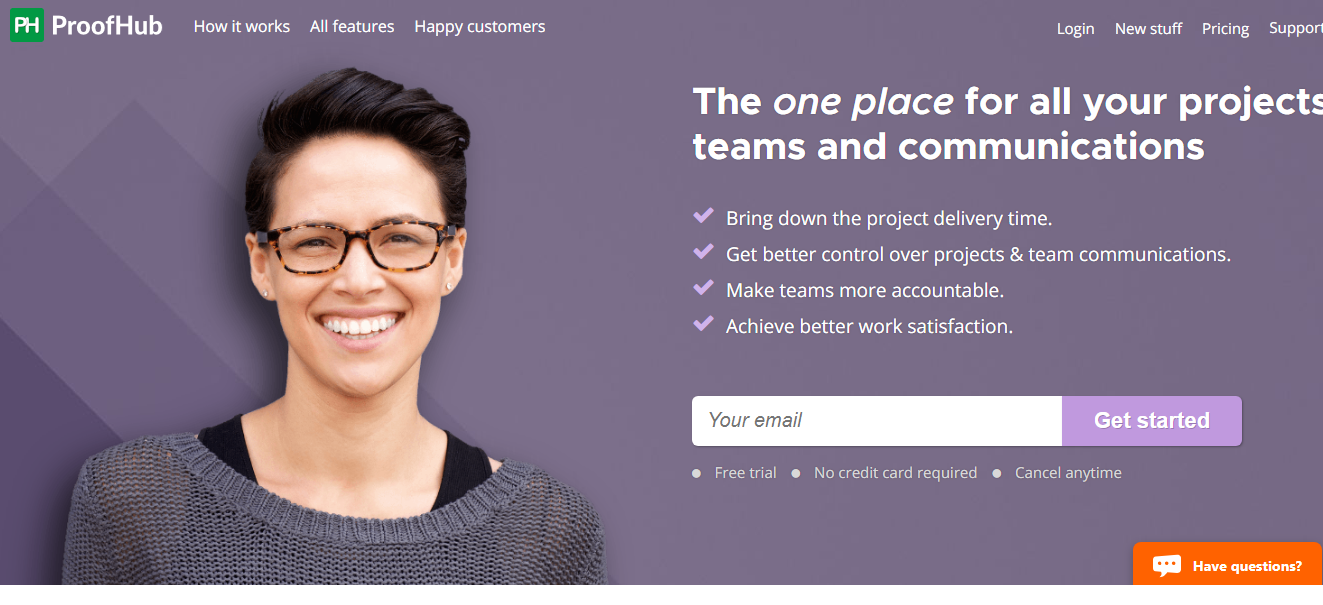The screenshot features the homepage of the Proofhub website. In the top left corner, the Proofhub logo is displayed inside a green box with the initials "pH." Adjacent to the logo, the website's navigation tabs read: "How It Works," "All Features," "Happy Customers." Further to the right, there is a substantial space before additional tabs: "Login," "New Stuff," "Pricing," and "Support."

In the main body of the webpage, an individual in casual attire is seen smiling warmly at the camera on the left side, adding a personal touch. To the right of this image, the headline "The one place for all your projects, teams, and communications" is prominently displayed. Below this is a detailed checklist highlighting the benefits of the site: "Reduce project delivery time," "Gain better control over projects and team communications," "Increase team accountability," and "Achieve higher work satisfaction."

An email input box invites users to enter their email addresses, accompanied by a "Get Started" button to initiate the sign-up process. The webpage also emphasizes a free trial with the phrases "No credit card required" and "Cancel any time."

In the bottom right corner, an interactive help option appears, indicating that users can "Have questions?" This section likely leads to a Q&A area, or allows interaction with an AI bot or a chat representative to obtain more information about Proofhub, its functionalities, and specific project needs.